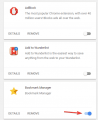The image is blurry and difficult to discern, but it features specific noticeable elements. It has a light gray border on all sides (top, left, right, and bottom). Within the image, there are three white rectangular sections, each separated by light gray areas. 

In the top rectangle, there is a gray and red logo positioned to the left, followed by some text on its right and beneath it. Below this segment, on the left side, are the words "details" and "remove," accompanied by a toggle switch that can be turned off.

The middle rectangle contains a red and blue logo on the left, with some text to its right and below it. Beneath this, there are the options "details" and "remove," along with another toggle switch that can be turned off.

In the bottom rectangle, there is a gold star on the left side, followed by some text on its right. Below this section, similar to the ones above, it says "details" and "remove." It also has a toggle switch, which is colored blue, indicating that it is turned on. Additionally, there is a red arrow pointing at this toggle switch.